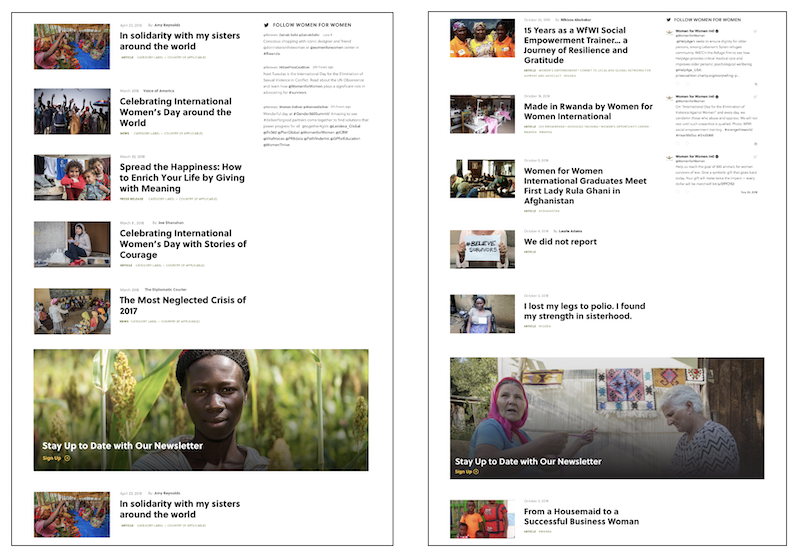The image consists of two side-by-side screenshots taken from a webpage, possibly from a website focused on women's issues. Each screenshot features a series of smaller images on the left, with six visible pictures in each feed and a larger, main image at the top, totaling seven images per column.

On the far left screenshot, the largest image highlights an African-American girl standing in a lush, green field. The overlaid text reads, "Stay up to date with our newsletter," followed by a "Sign up" button. 

The screenshot on the right showcases a different main image. This time, two women are featured; one appears to be holding an object, perhaps indicating they are engaged in crafting rugs. The same newsletter prompt, "Stay up to date with our newsletter," is accompanied by a "Sign up" button. 

At the top of both screenshots, text encourages visitors to "follow Women for Women," suggesting this could be the name of the website. Below this header, various article titles are visible:
- "In solidarity with my sisters around the world"
- "Celebrating International Women's Day around the world"
- "Spread the happiness: How to enrich your life by giving with meaning"

These articles cascade down the page, emphasizing themes of solidarity, celebration, and meaningful giving among women globally.